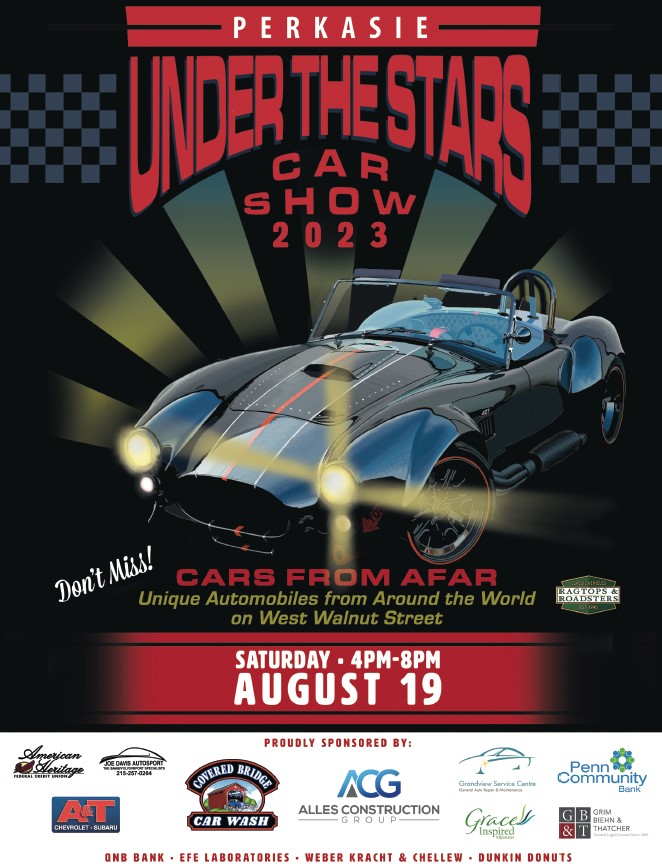The digital image is an advertisement flyer for the "Perkasie Under the Stars Car Show 2023." The background predominantly features black, accented with a checkered blue and black pattern at the top. There is a vibrant red banner across the top with bold, white text spelling out "P.E.R.K.A.S.I.E.," and just below it, in red letters, "Under the Stars Car Show 2023." 

Centrally displayed is a detailed illustration of a classic, dark gray Porsche-type sports car, possibly from the 1930s or 40s. The car, a convertible, is oriented to the left with its headlights on, emitting beams of light. The car appears polished and pristine, symbolizing the elegance of the event.

Underneath the car, in prominent white text on a red background, is the exclamatory phrase "Don't Miss!" This is followed by, in red text, "Cars from Afar, unique automobiles from around the world on West Walnut Street." Further details, in the same white text on a red background, announce the event's timing: "Saturday, 4 p.m. to 8 p.m., August 19th."

Towards the very bottom, the flyer lists logos of the sponsors, beneath the heading "Proudly Sponsored By," which includes various businesses and car washes like A.T. and Covered Ridge Car Wash. Additionally, there is a specific logo for "Ragtops and Roadsters" to the right side of the image. Golden-green bursts of light add a festive touch, enhancing the flyer’s allure.